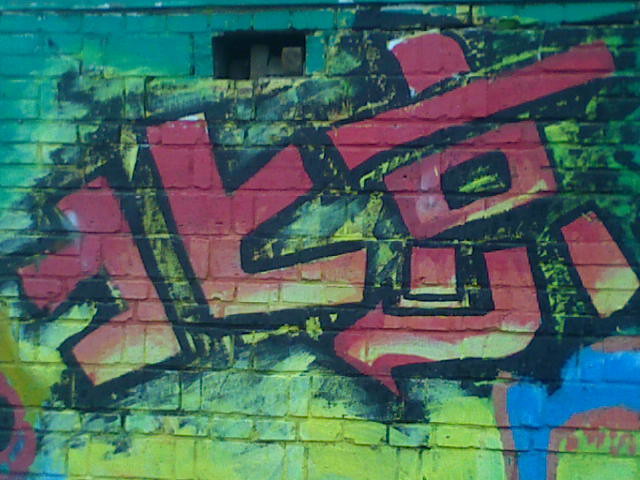This close-up photograph captures a graffitied brick wall teeming with vibrant, varied colors. Dominating the wall are characters that appear to be Chinese or Japanese, rendered predominantly in red, outlined in black, with yellow accents at the bottom. Amidst the characters, a red arrow points to the left. The graffiti sprawls across the textured backdrop of the bricks, smudging together in hues of green, blue, and yellow, interspersed with random black patches, giving a somewhat gritty appearance. A notable feature is a brick missing at the top, slightly to the left. The absence of any people, text, or watermarks keeps the focus solely on the graffiti and the texture of the aged wall. The photograph, slightly wider than it is tall, presents a vivid and detailed snapshot of urban street art.